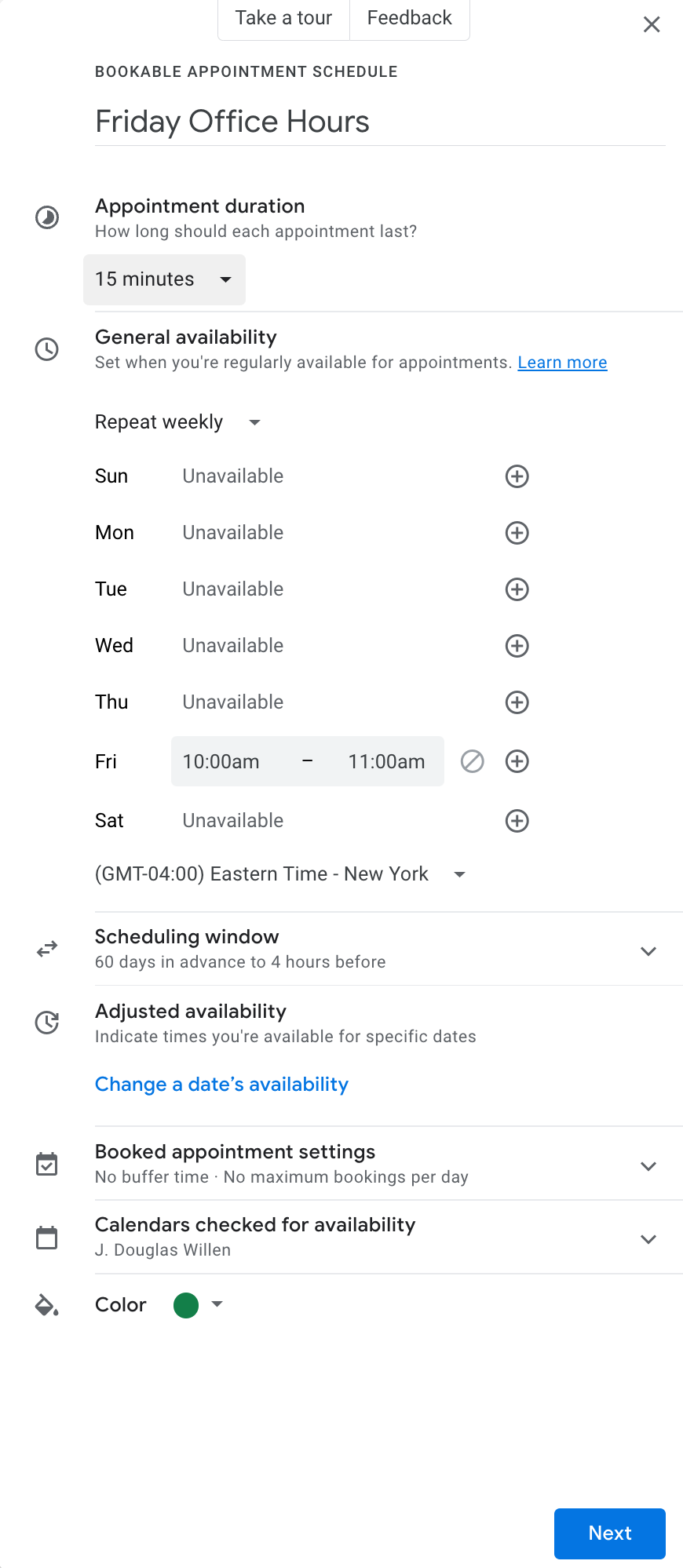The web page features a clean, white background at the top with two buttons labeled "Take a Tour" and "Feedback." A small box with an "X" allows users to close this section. Below, in black text, it reads "Bookable Appointment Schedule" with "Friday Office Hours" specified.

A circular icon with a line beside the phrase "Appointment Duration" prompts users to specify the length of each appointment. A light blue dropdown box set to "15 minutes" includes a down arrow for adjusting the time. Another circular icon featuring a clock introduces the "General Availability" section, instructing users to set their regular hours for appointments.

A blue, underlined "Learn More" link provides additional information. The "Repeat Weekly" option includes a dropdown menu. Days of the week are listed, showing availability statuses: 
- Sunday: Unavailable (circle with a plus)
- Monday: Unavailable (circle with a plus)
- Tuesday: Unavailable (circle with a plus)
- Wednesday: Unavailable (circle with a plus)
- Thursday: Unavailable (circle with a plus)
- Friday: 10:00 AM to 11 AM (circle with a slash and a plus)
- Saturday: Unavailable

Further down, "GM" is noted at "4 o'clock Eastern Time, New York." The "Scheduling Window" section features a left-aligned icon, while "Adjusted Availability" is indicated with another clock icon. 

In blue text, the option "Change Dates Availability" appears. A calendar icon with a check mark symbolizes "Booked Appointment Settings," where calendars synchronize for availability indicated by a green circle. A "Next" button concludes this section.

This organized layout facilitates efficient appointment management through clear visual cues and intuitive navigation options.